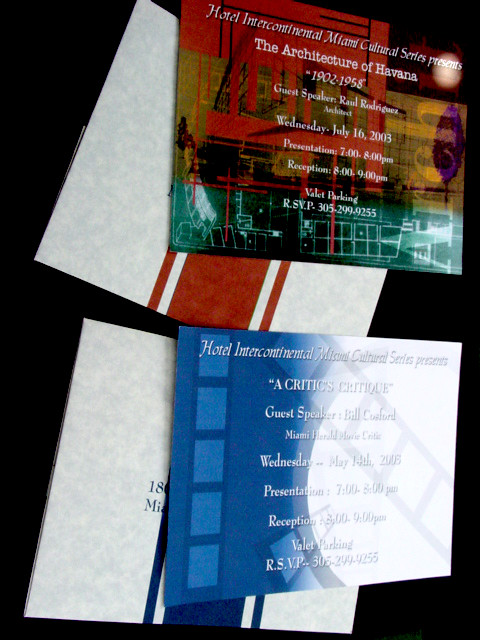The image depicts a black board adorned with various postcards and flyers of different colors. The most prominent flyer advertises the "Hotel Intercontinental Miami Cultural Series Presents: The Architecture of Havana, Havana, Cuba, 1902 to 1958." This event features a presentation by guest speaker and architect Raul Rodriguez. It occurred on Wednesday, July 16, 2003, from 7 to 8 p.m., with a reception following from 8 to 9 p.m. The flyer notes the availability of valet parking and provides an RSVP contact number.

Another visible flyer, albeit less clear due to a camera flash and slightly blurred text, also advertises an event under the Hotel Intercontinental Miami Cultural Series. This second event is titled, "A Critic's Critique," featuring guest speaker Bill Crawford and mentions "Miami, Hell Road." Both flyers share similar design elements, such as color tinting and collage-style imagery of buildings, with the main flyer portraying an old, color-tinted photograph of a hotel.